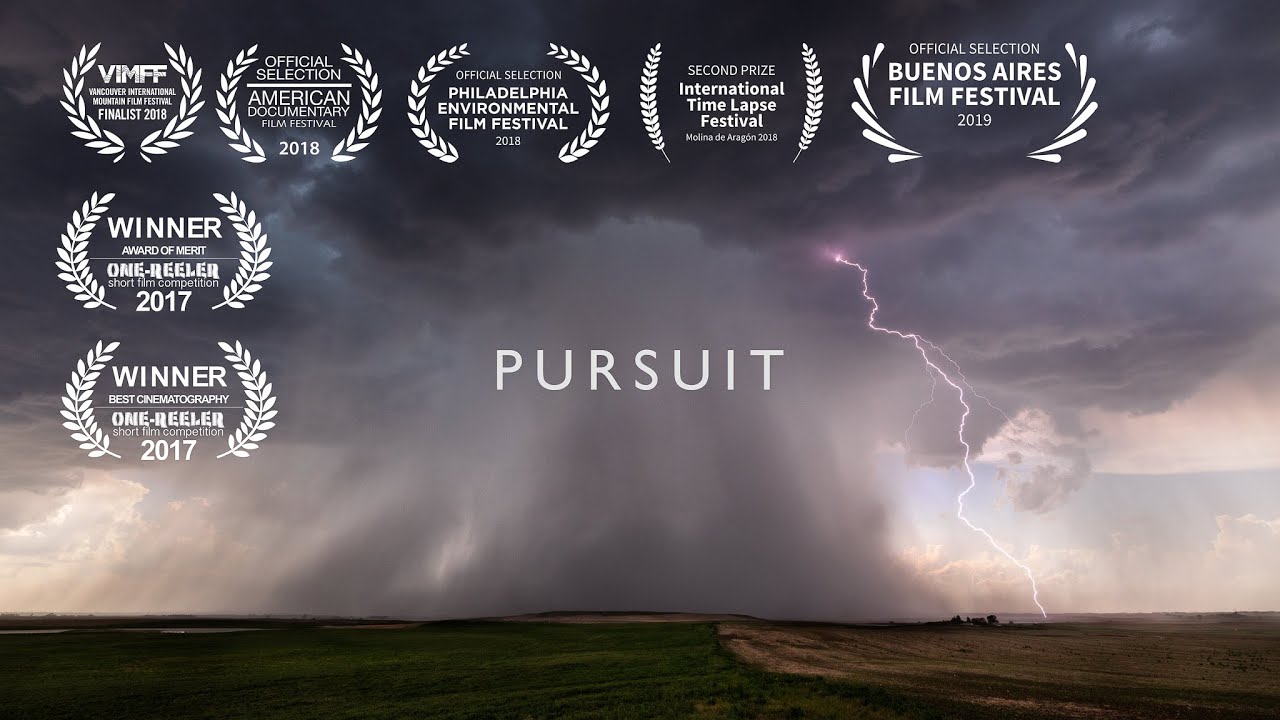This image appears to be a dramatic, wide-format movie poster or thumbnail for a YouTube video, presenting a gripping scene where a massive tornado dominates a flat, farmland landscape. The sky, filled with dark, menacing storm clouds, transitions from black at the top to lighter grays and blues near the horizon. In the distance, a vivid lightning bolt strikes the ground to the right of the swirling tornado. Central to the composition, bold white capital letters spell out "PURSUIT." Surrounding the title are seven distinctive award emblems, featuring prestigious recognitions from various film festivals such as "WINNER Best Cinematography 2017," "WINNER Award of Merit 2017," and official selections from the "American Documentary Film Festival 2018" and "Buenos Aires Film Festival 2019." Each award is encircled in delicate leaf or flower designs, adding a touch of elegance to the ominous and powerful scene.